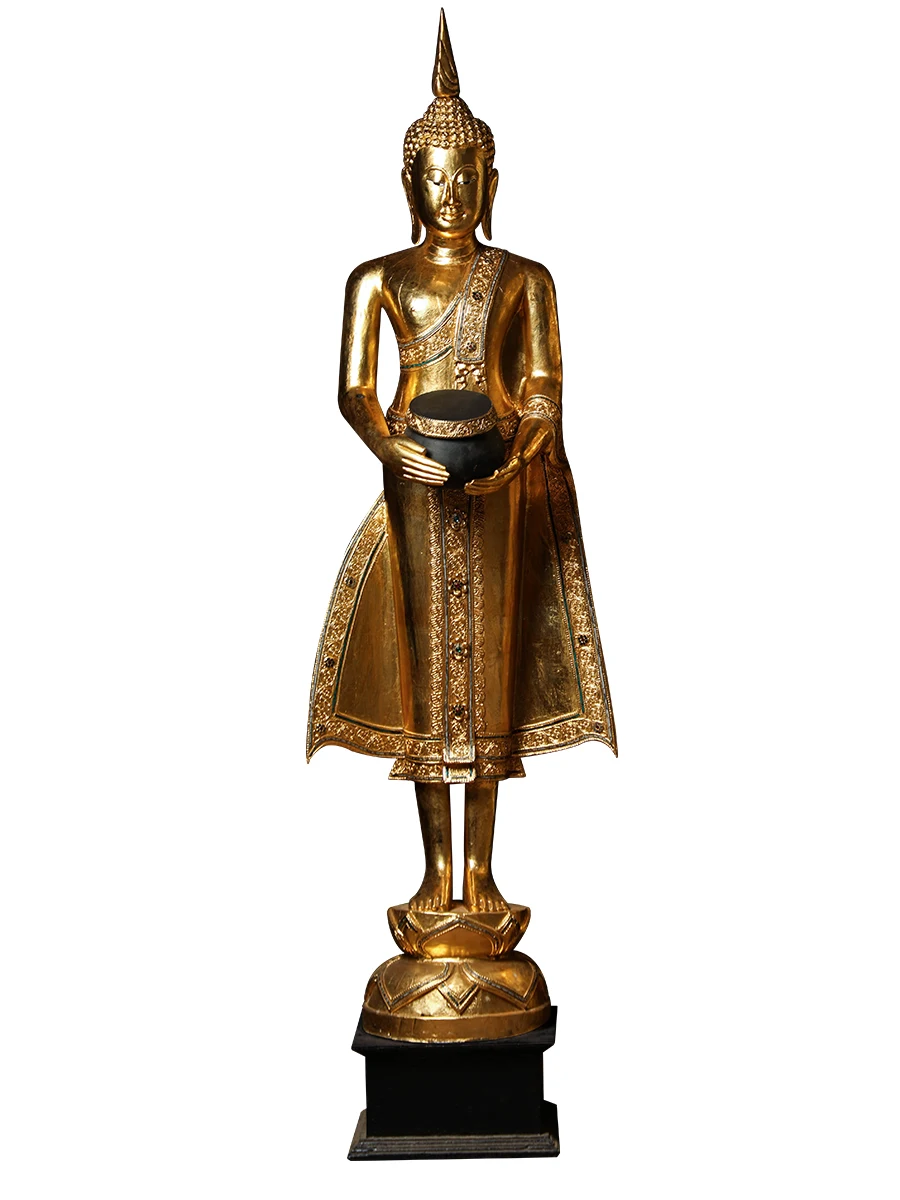The image depicts a detailed bronze or brass statue standing on a black pedestal. This ornamental figure, likely representing a religious or Buddhist symbol, is positioned at the center of the white background. The statue features a human-like figure with a slender body, adorned in a dress-like robe and a cape lined at the edges. The figure wears a striking pointy hat resembling a helmet or a unicorn horn. The statue's hands are extended outward, holding a black pot with a gold band encircling its top. The bronze or brass statue showcases the figure wearing platform shoes, though some descriptions suggest bare legs colored gold from the knees down. The figure stands on an upside-down half-circle base, further elevated by a black square platform.